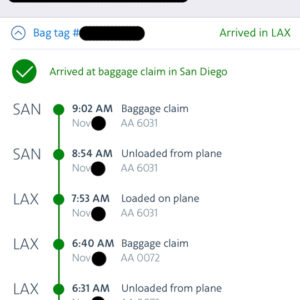Here is a cleaned-up and detailed caption for the described image:

---

"Screenshot of a travel information document with a white background and a gray header bar at the top. The document consists of two main columns. The left side features a blue text label reading 'Bag Tag Number,' though the actual number is obscured by black. Below this is a green text reading 'Arrived in LAX.' The right side of the document provides a detailed itinerary, highlighted by a prominent green check mark within a green circle, accompanied by the text 'Arrived at Baggage Claim in San Diego.'

Further down, the itinerary details multiple segments of a travel journey:

1. 'San' at 9:02 AM - November (exact date hidden), marked with flight number AA6031.
2. Next, 'San' at 8:54 AM - Unloaded from train.
3. 'LAX' at 7:53 AM - Loaded on plane.
4. 'LAX' at 6:40 AM - Baggage Claim.
5. 'LAX' at 6:31 AM - Unloaded from plane.

It appears there are five different connections, indicating a complex travel path involving stops at San Diego (SAN) and Los Angeles (LAX). Specific dates are obscured by black circles, making it unclear when these events occurred."

---

This description provides a detailed and clear understanding of the visual content and layout of the travel document.